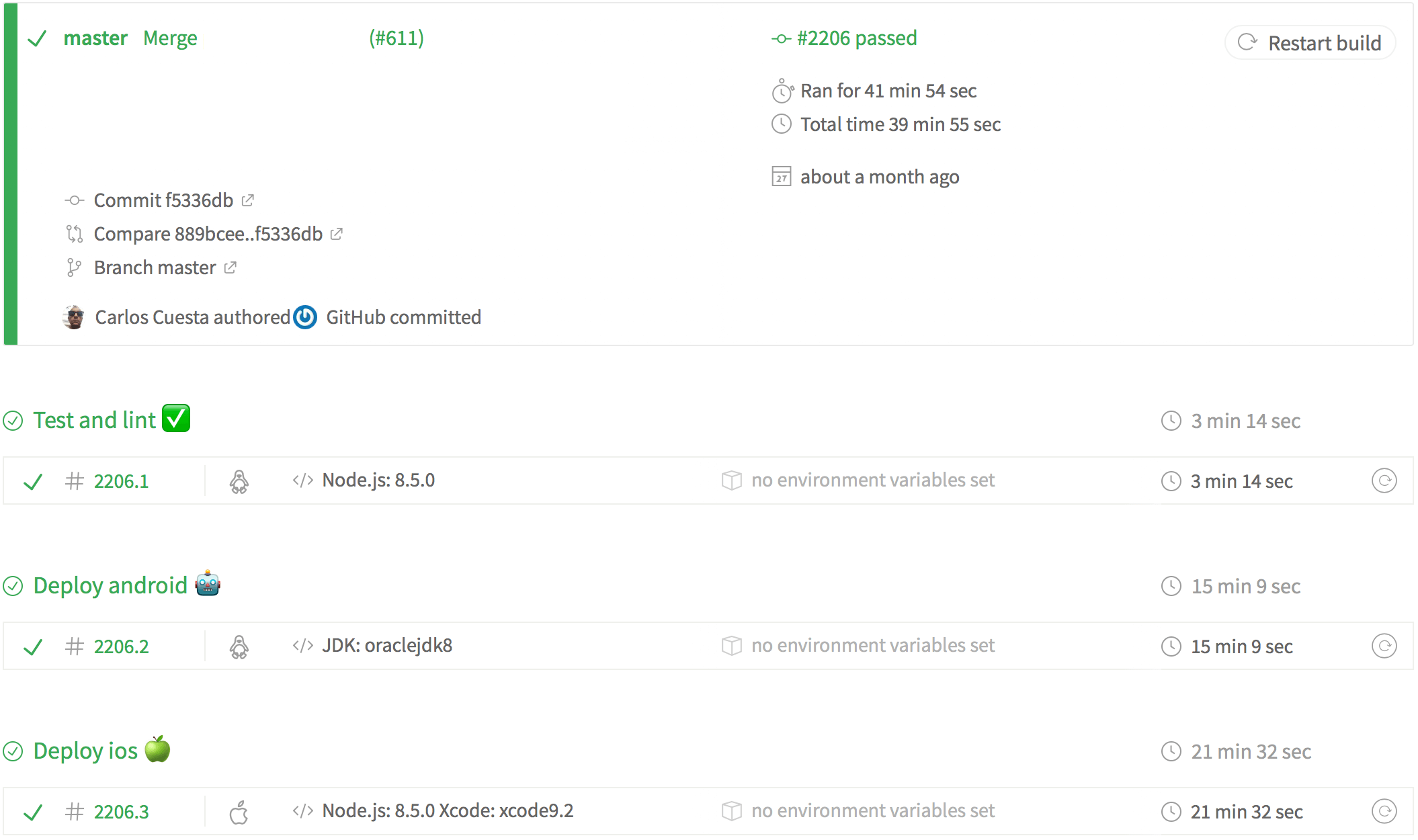This screenshot captures a detailed view of a technical program interface, likely related to a continuous integration/continuous deployment (CI/CD) pipeline. The background is white, accented with green and black elements for various indicators and text.

### Upper Left-Hand Corner:
- A green vertical bar drops halfway down the screenshot.
- Adjacent to the bar, a green checkmark is featured next to the text "Master Merge."

### Upper Right-Hand Corner:
- A "Restart Build" button with a refresh symbol.

### Middle Section:
- To the right of "Master Merge," a label reads "#611."
- Below that, another label displays "#2206 Passed."

### Textual Details:
- Key commits and comparisons are listed:
  - "Commit F5336DB" with a pop-up symbol.
  - "Compare 889BCEE..F5336DB" with another pop-up symbol.
  - "Branch Master" with an additional pop-up symbol.
  - Authored by "Carlos Cuesta."
  - GitHub logo followed by "GitHub committed."

### Additional Information:
- Under "#2206 Passed," more descriptive text includes:
  - "Ran for 41 minutes 54 seconds."
  - "Total time 39 minutes 55 seconds."
  - Conducted "about a month ago."

### Left Side Columns:
Three distinct columns detail various build processes:
1. **Test and Lint** (with a checkmark):
   - #"2206.1 node.js..8.5.0" with "No environment variable set," duration of 3 minutes 14 seconds.
2. **Deploy Android** (indicated by a robot icon):
   - #"2206.2 JDK Oracle JDK 8" with "No environment variable set," duration of 15 minutes 9 seconds.
3. **Deploy iOS** (indicated by an Apple symbol):
   - #"2206.3 node.js 8.5.0 Xcode..Xcode 9.2" with "No environment variable set," duration of 21 minutes 32 seconds.

This comprehensive image encapsulates various stages of a CI/CD pipeline, complete with timestamps, environment details, and commit metadata, set against an intuitive user interface design.